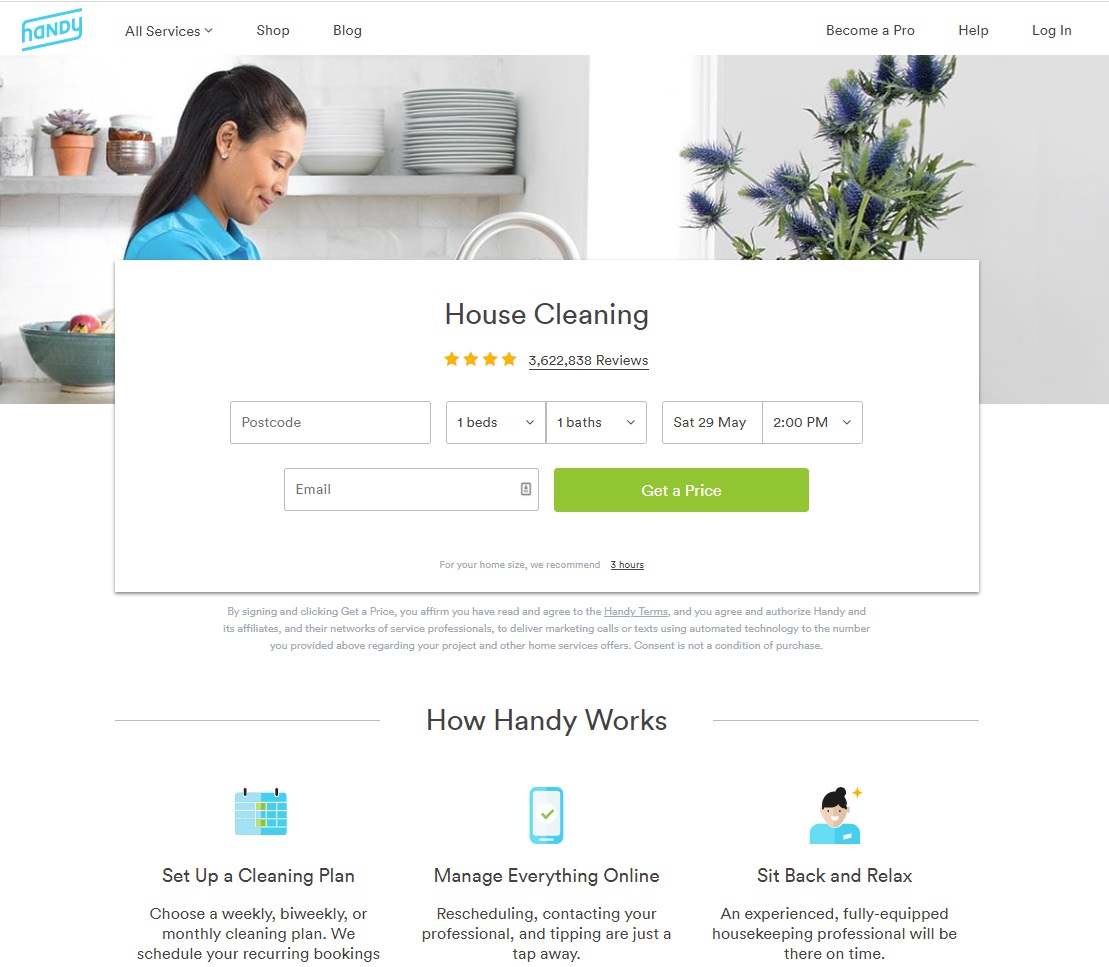In the image, the top left corner prominently features the word "Handy" written in blue. To the right of this logo, there are three tabs labeled "All Services," "Shop," and "Block." On the top right of the image, another set of three tabs appear: "Become a Pro," "Help," and "Login," all written in black against a white background.

Dominating the central portion of the main page is a headline that reads "House Cleaning," accompanied by a yellow four-star rating based on 3,622,883 reviews. Below this, there are interactive fields for users to input their postcode, select the number of bedrooms and bathrooms, choose the date and time for service, and enter their email address. Adjacent to these fields is a prominent green button labeled "Get a Prize."

Underneath these main fields, there's a recommendation suggesting that for a home of average size, 3 hours of cleaning is advisable. Following this, a disclaimer states: "By signing and clicking 'Get a Prize,' you affirm that you have read and agree to the Handy terms and you agree and authorize Handy and its affiliates and the NHLG service providers to deliver marketing calls or texts using automated technology to the number you provided above regarding your project and other home services offers. Contact is not a condition of purchase."

At the bottom of the image, a section titled "How Handy Works" presents three steps or options. The first option, located on the left, advises users to "Set up a cleaning plan," offering choices for weekly, bi-weekly, or monthly plans, and noting that Handy schedules recurring bookings. The middle option highlights the convenience of managing all aspects of the service online, including scheduling, contacting professionals, and tipping. The final option on the right encourages users to "Sit back and relax," promising that fully-equipped housekeeping professionals will arrive on time to provide service.